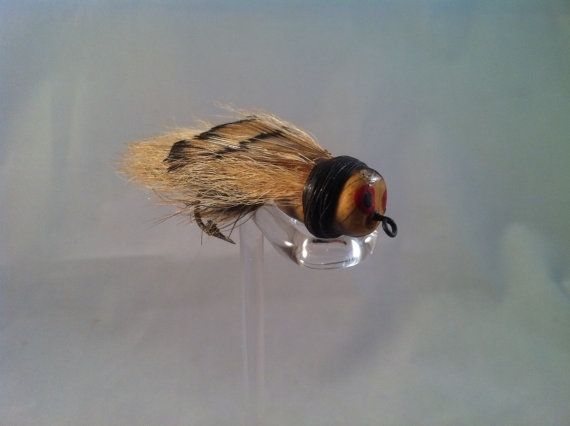This image depicts a close-up photograph of a homemade fishing fly, meticulously crafted to resemble a stinging insect. The fly is centrally placed on a translucent pedestal against a gray background, with the craftsmanship intricately highlighted. The fly features a prominent gray hook at the bottom, curled under its body, and another hook at the right side where black string is tightly wound around a wooden knob forming the head. The head is detailed with amber coloring, large brown eyes, and what looks like a hooked antenna or nose. A black band separates the head from the bushy tail, which is made of animal fur colored in shades of brown with black stripes, enhancing its insect-like appearance. The body is oval-shaped with light brown, furry wings, and a dark gray pointed stinger-like projection under its hind part. Two curled, white forelegs are also present, adding to the lifelike design of this fishing lure.